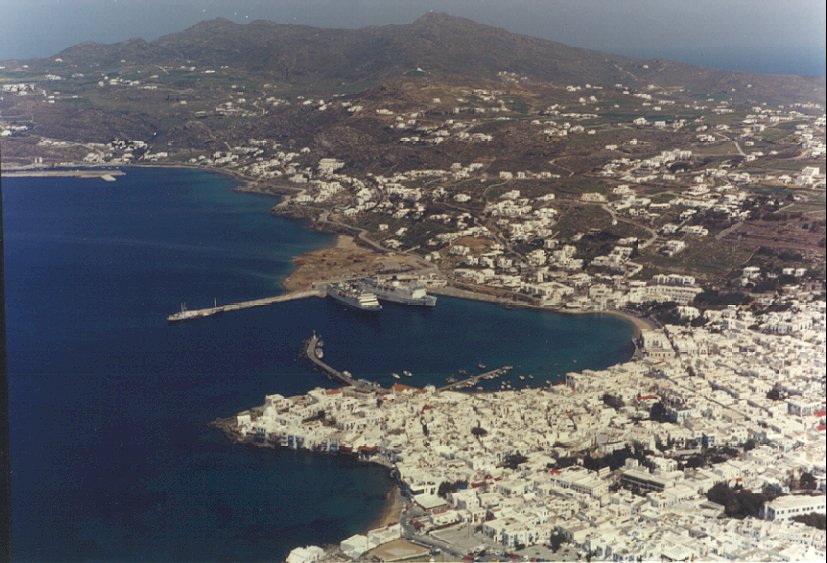This is an overhead, aerial view of a coastal port area, likely taken from a height of 1,000 to 1,500 feet. To the left of the image stretches a vast, deep blue body of water, possibly an ocean or large lake. Two large ships are moored along a dock that extends into the water, slightly larger than small boats but smaller than large yachts. In the foreground, a dense cluster of white houses and buildings tightly populate the bottom right section, giving way to a more sparse arrangement of similar white stone and brick structures as the view extends upward. Hills, which are brown and green with patches of trees, frame the background, while a hazy, dark sky looms above. The landscape appears lush and rugged, resembling an isthmus or a coastal city with a mountainous terrain.